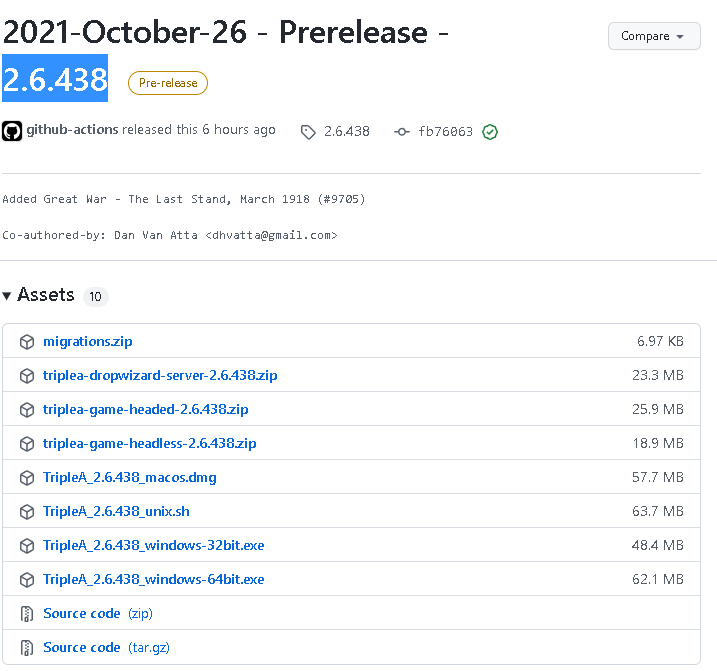This image is a cropped screenshot of a GitHub pre-release page. The background at the top is white, and it features a digital-type font. Prominently displayed in very large black letters is the text "2021 October 26 Pre-release." Below this heading, towards the left, it shows the version number "2.6.438," which is highlighted with a blue rectangle. To the right of the version number, there is a yellow bubble that reads "pre-release."

At the bottom of the top banner, in gray font, it states, "GitHub Actions released this six hours ago." To the right of this message, there is a tag icon, next to which the version number "2.6.438" is repeated.

Further down, the text "Added Great War: The Last Stand March 1918. Co-authored by Dan Adda" is displayed, with Dan Adda's email address positioned to the left. All this text is in gray font.

Towards the left side of this section, the word "assets" is presented in large digital font. There is an expanded drop-down box to the left of this text, and to its right, a gray bubble with the number "10" inside indicates the number of assets listed. The box below "assets" displays the names of 10 files on the left, with their respective sizes shown on the far right.